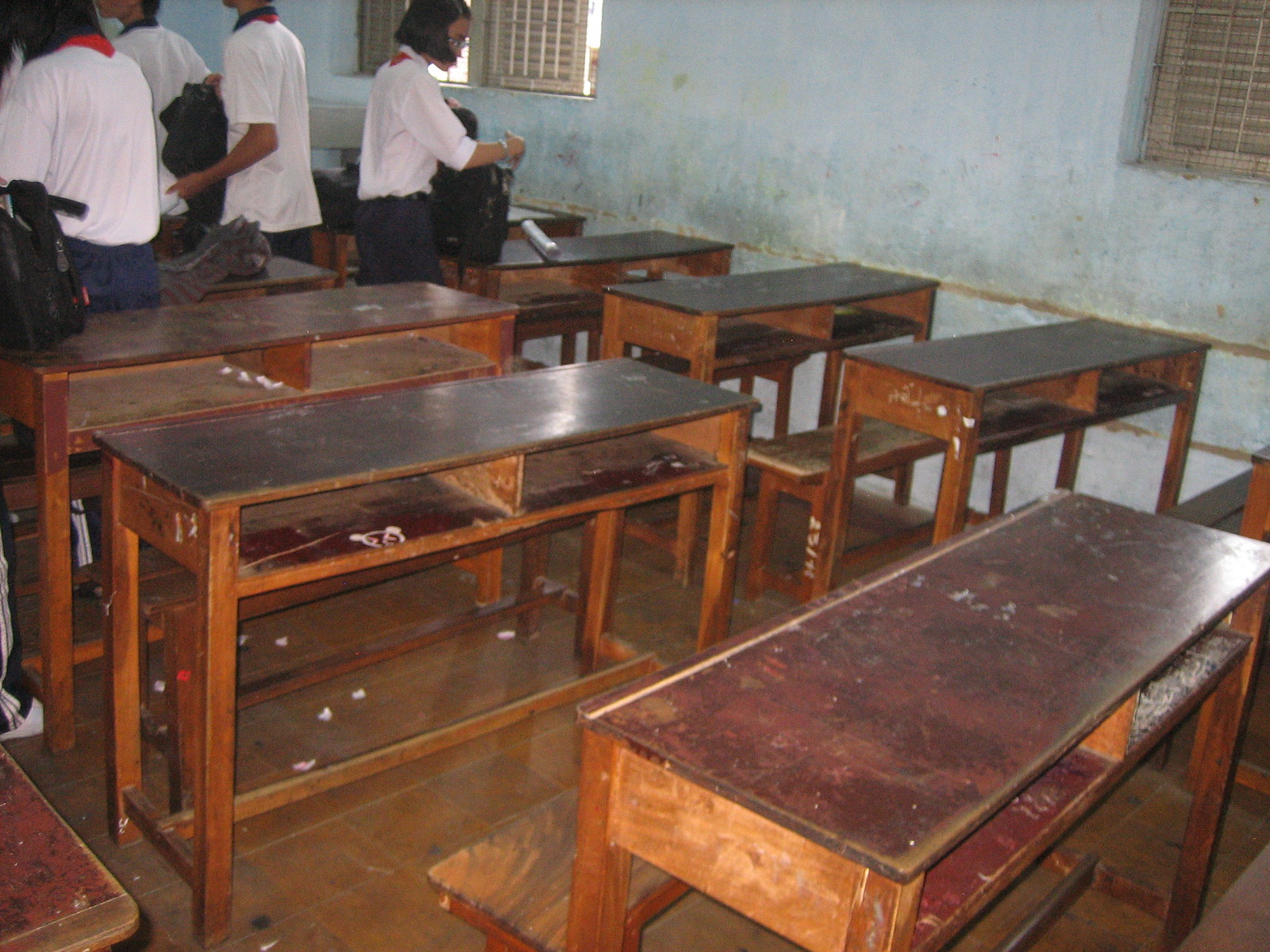The image depicts the interior of a dilapidated classroom, likely located in a third-world country, possibly in Asia. The room features worn wooden desks, each capable of seating two students, with two small rectangular cubbies inside that have been scratched, chipped, and written on over time. Behind each desk is an equally worn wooden bench. The classroom's concrete walls, painted a fading blue, are dirty and show signs of deterioration. Windows with broken grates allow light to filter through. The brown wooden floor is covered with debris. In the upper left corner, four students, likely Asian, are seen wearing white shirts, blue pants, and red ties, possibly part of a school uniform. They appear to be loading items into their book bags. The overall atmosphere suggests an environment that has endured much use and hardship.